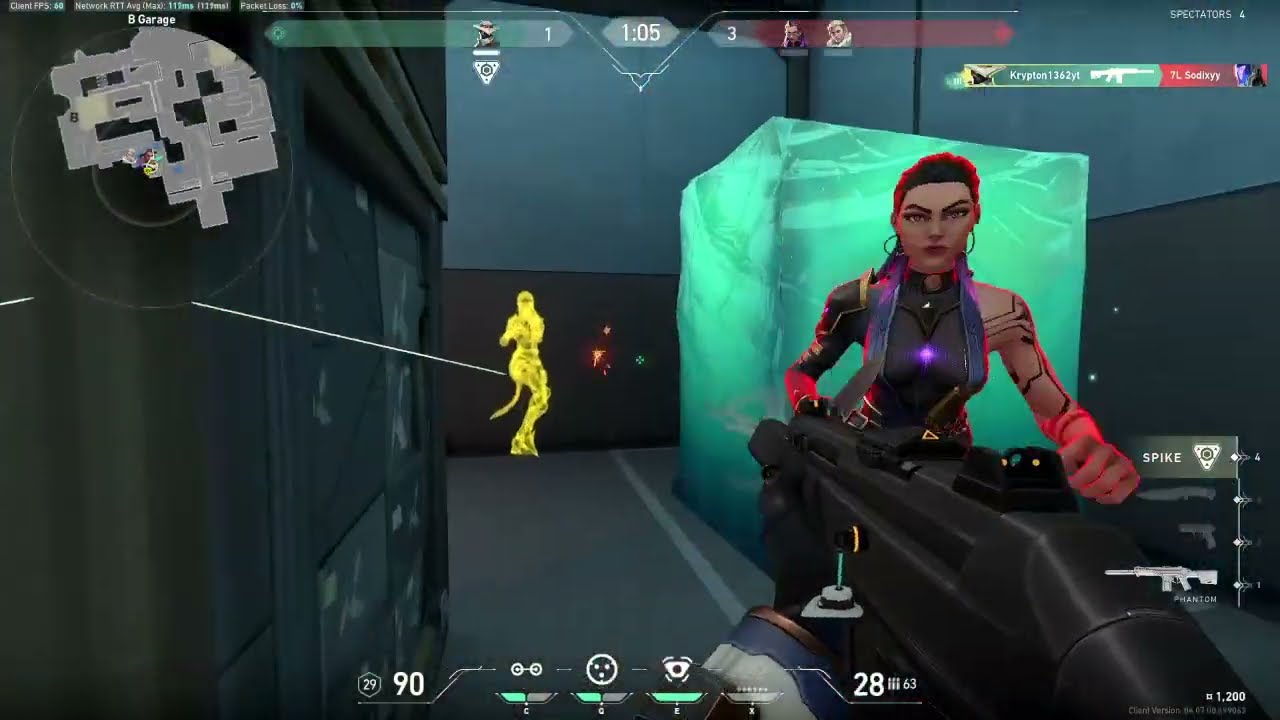This screenshot from a first-person shooter video game showcases a vivid, futuristic environment. Dominating the scene is a female character positioned slightly off-center to the right, donned in black and purple armor with glowing red accents on her hands. Her outfit clings tightly to her form, showing off intricate tattoos and a black sleeve on her right arm. She has brown hair, hoop earrings, and dark eyes. The character is wielding a large black gun that stretches from the middle of the image to the lower right corner, giving a close-up view of the weapon.

In the background, the setting appears to be a high-tech, space-themed computer room with a mixture of dark gray, blue, and black tones. A large, glowing green cube illuminates the left part of the image. To the left of the main character, an outline of another female figure, highlighted in yellow, stands with a tail-like feature, indicating a potential target. The upper left corner features a gray-toned map, while various user interface elements such as health bars, ammo count, and other typical FPS indicators (like 'spike' and the numbered and lettered commands 'C, Q, E, X') populate the screen. A time display reading '1:05' and icons of additional characters, including a man and a woman, can be seen at the top. This richly detailed scene captures the intensity and complexity of the gameplay environment.